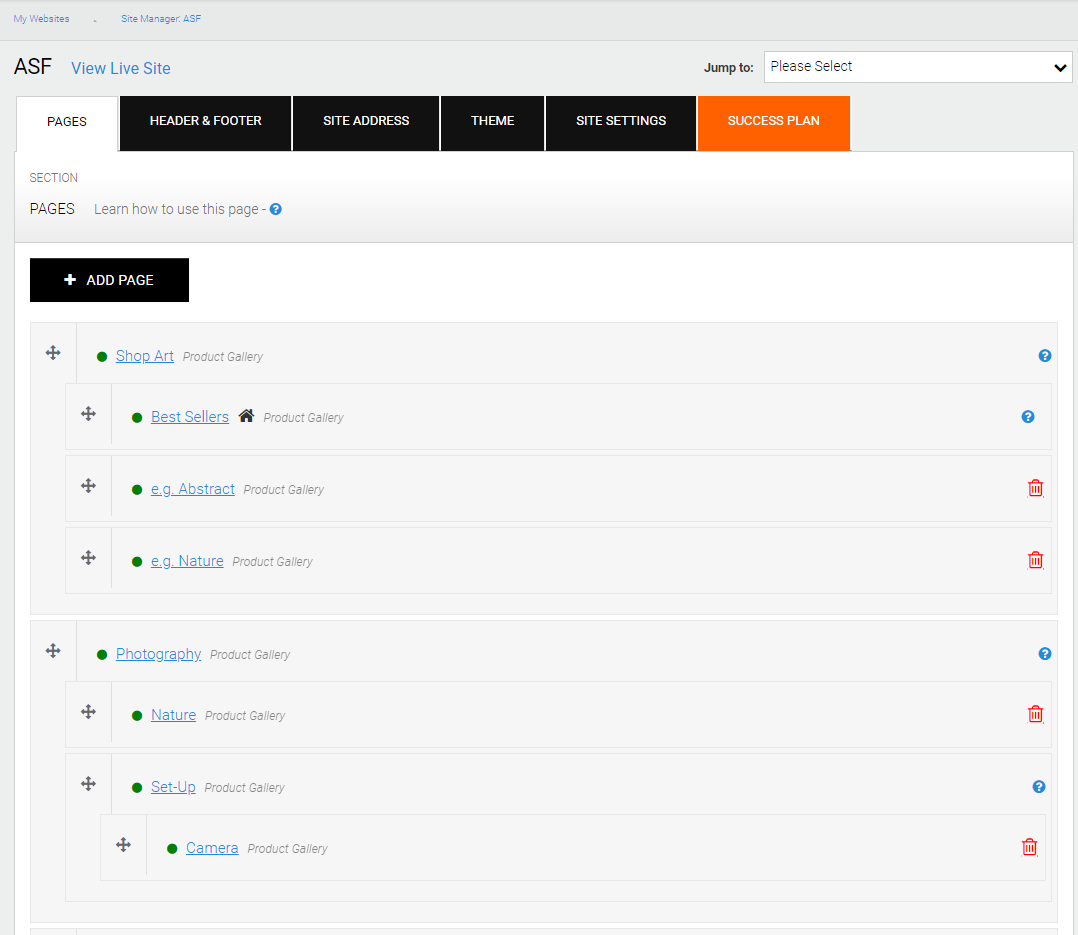The image depicts a website's user interface, organized for site management. At the top right, the phrase "Jump to" is displayed, followed by a small rectangular section labeled "Please select" with an accompanying dropdown arrow, suggesting options can be expanded. In the top left corner, the text "My Websites" is shown in blue, with "Site Manager ASF" situated to its right, also in blue.

Central to the image, slightly left-aligned, is a prominent black rectangle featuring white text that reads "Add Page" alongside a white plus symbol. Below this section, there are eight green bullet points, each representing a page or section on the website. They are listed in the following order: "Shop Art," "Best Sellers," "EG Abstract," "EG Nature," followed by a new row containing "Photography," "Nature," "Setup," and "Camera." Adjacent to the words "Abstract," "Nature," and "Camera" on the far right, a small red trash icon is visible, indicating options for deletion.